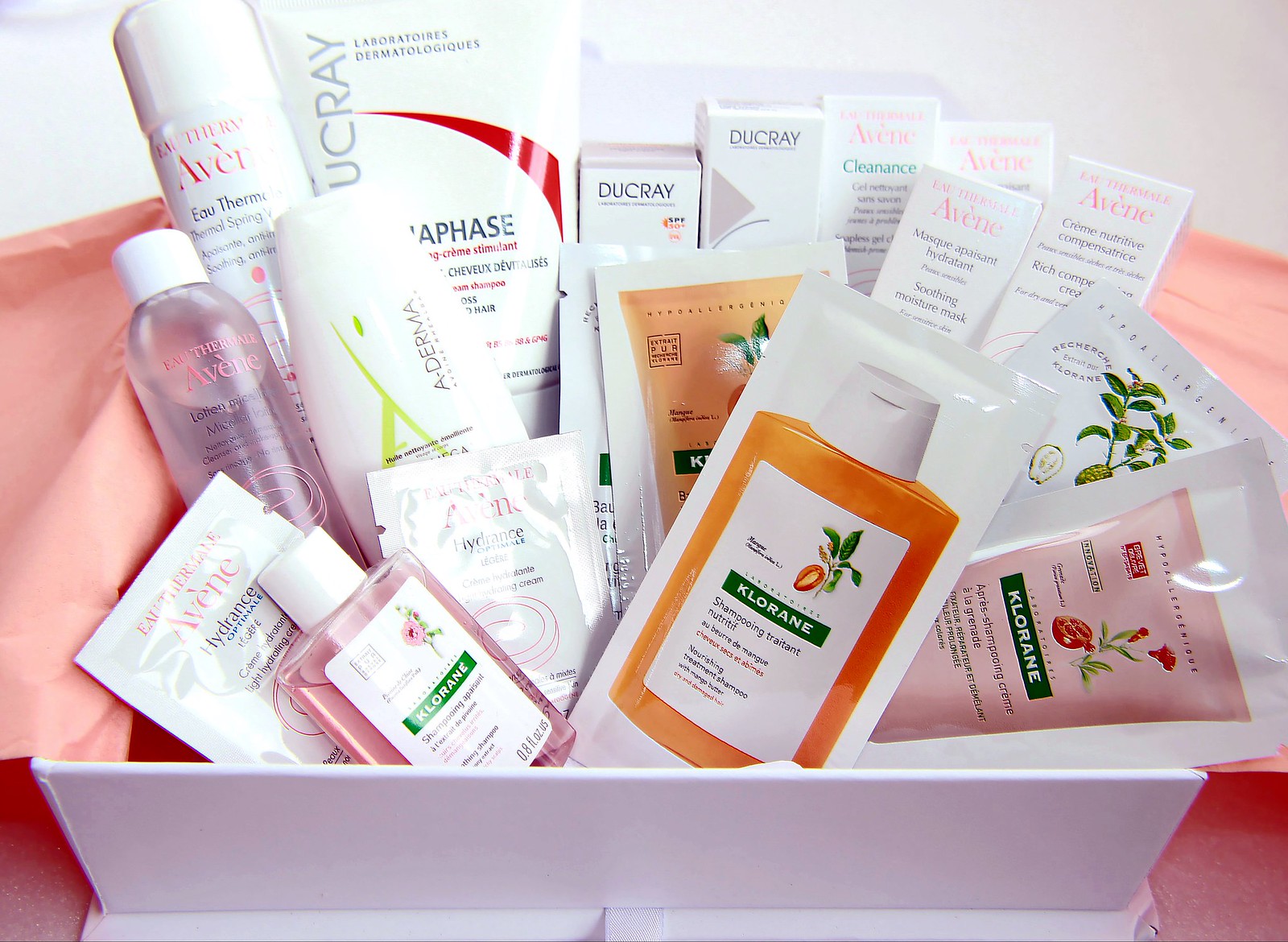This image showcases a meticulously arranged toiletry gift set, predominantly featuring a purple and pink color scheme. The set is displayed on a pinkish surface, with apricot-pink tissue paper providing a soft backdrop. The assembly of this display suggests it is intended as a thoughtful gift. 

At the forefront, there is a sachet labeled "Shampooing," although the rest of the text is obscured, indicating it might be a shampoo or wash product. Several other product sachets are also visible. A small plastic container with a white cap is nestled among them, along with additional small sachets.

A bottle containing a clear liquid, possibly toner, also with a white cap, stands beside a larger white tube. Another significant product is a large tube adorned with red text, partially readable as "phase." This tube is the most prominent item in the set. Additionally, a dispenser resembling those used for shaving cream is included.

Towards the back, there are six small boxes, each containing products, completing the gift set. The entire arrangement is thoughtfully curated, making it an ideal present for someone special.